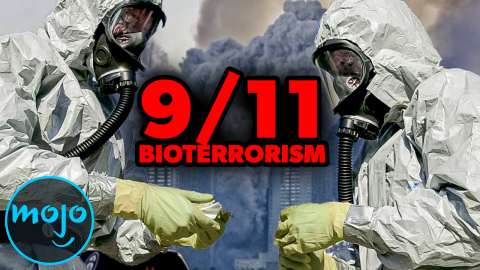The poster prominently features two men in full hazmat suits, including heavy-duty yellow gloves, black gas masks with clear visors, and protective shields, all suggesting protection from bioterrorism. They appear to be working under a hood likely connected to a ventilation device such as a Scott Air Pack. Dominating the center of the poster are the large red letters "9-1-1," with the word "BIOTERRORISM" in all caps directly beneath, both in a 3D effect with black borders. Off to the bottom left, there's the Mojo logo—a circle filled with a dark, translucent color, featuring "Mojo" in light blue-green lettering and a smiling face under the "J." The background is a haunting scene of the 9-11 aftermath, filled with tremendous smoke rising against a white sky, reminiscent of the city's skyline and the collapsed Twin Towers.